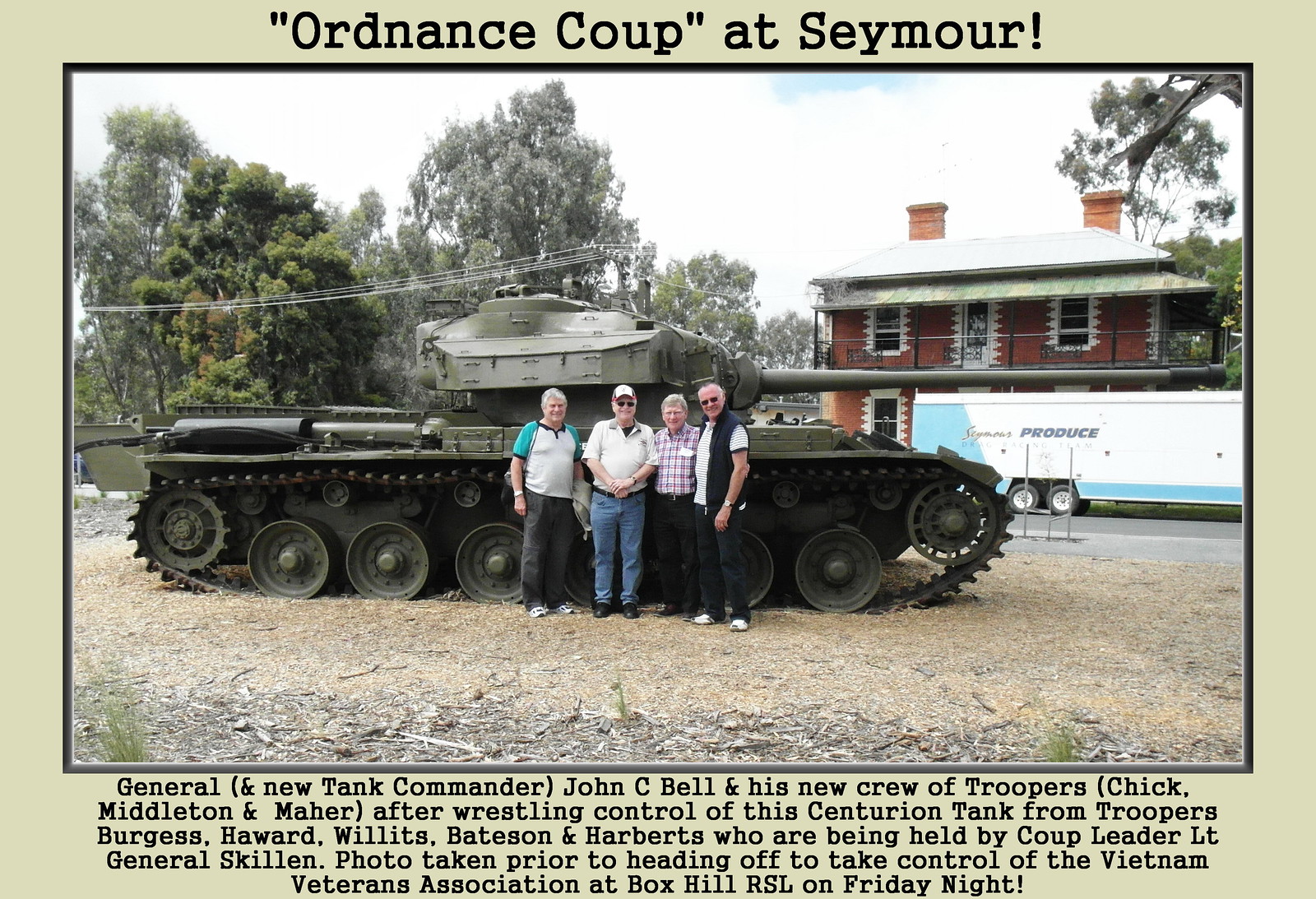The photograph features four elderly men, likely in their 70s or 80s, standing in front of a formidable olive-green Centurion tank. This substantial piece of military machinery is set against a backdrop of a vivid blue sky with white fluffy clouds, tall green trees, and the brown mulch on the ground. To the right of the tank, there's a colorful van that's purple, light blue, and predominantly white with a sign indicating something about produce. Behind the group, a house with a white roof, two reddish-brown chimneys, and white-trimmed windows adds further detail to the setting.

The photograph is framed by a tan-colored thick border with a thin dark gray inner line. At the top of this border, black text reads "Ordnance Coup at Seymour." The bottom of the border provides additional context: "General and new tank commander John C. Bell and his new crew of troopers Chick Middleton and Marr, after wrestling control of the Centurion tank from Troopers Burgess, Howard, Willits, Bateson, and Harberts, who are being held by coup leader Lieutenant General Skillen. Photo taken prior to heading off to take control of the Vietnam Veterans Association at Box Hill RSL on Friday night." The four men in the photo are posed confidently in front of the tank, preparing for their mission.